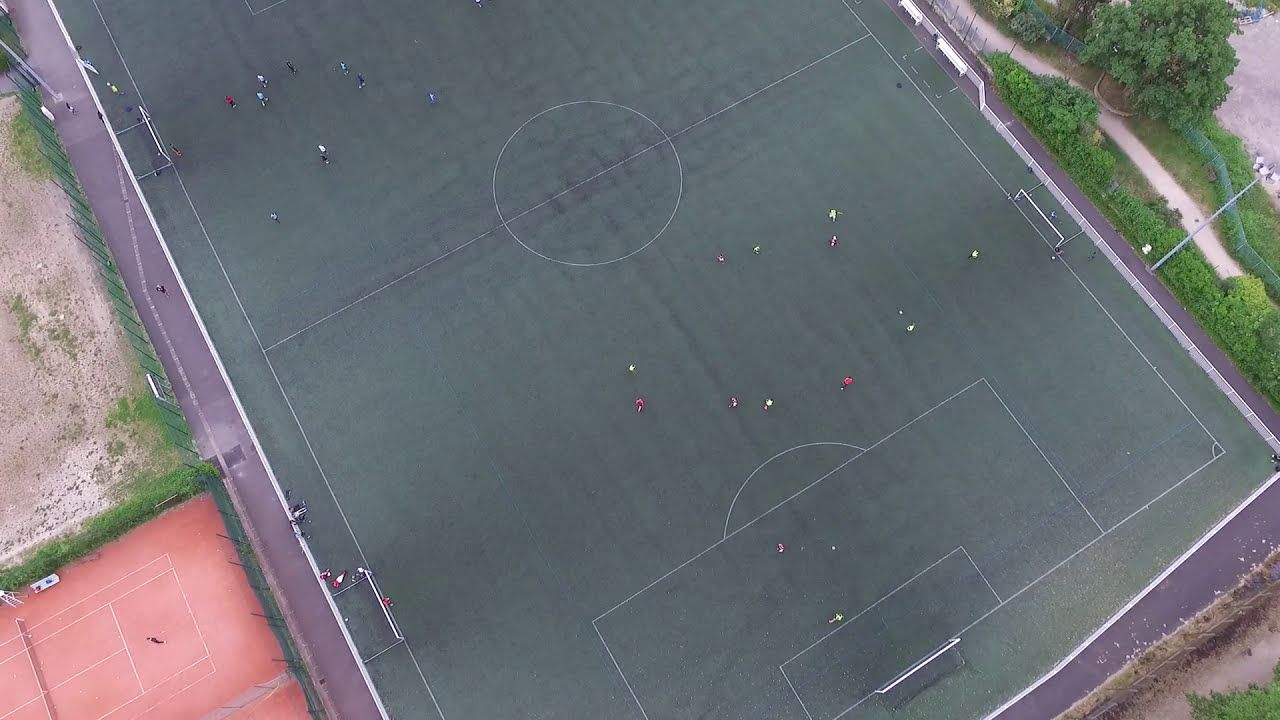This image is a high-angle, bird's-eye view shot, likely captured from a drone, looking directly down at a full-size soccer field surrounded by a black pavement walkway. The deep green AstroTurf field is adorned with white lines marking the goals and center. Dotted with tiny figures resembling colored specks, the players in red, yellow, blue, and black jerseys appear to be engaged in what seems like practice sessions, as opposed to a single game, due to the multiple setups. To the left of the soccer field, a salmon-colored clay tennis court stands out, occupied by a single player in dark clothing. Adjacent to the tennis court is a patch of bare dirt with sporadic grass growth. In the upper right, a cement trail meanders through a grassy area, flanked by trees on both sides. The height of the shot amplifies the minute appearance of the people, making every detail on the ground look remarkably small and intricate.